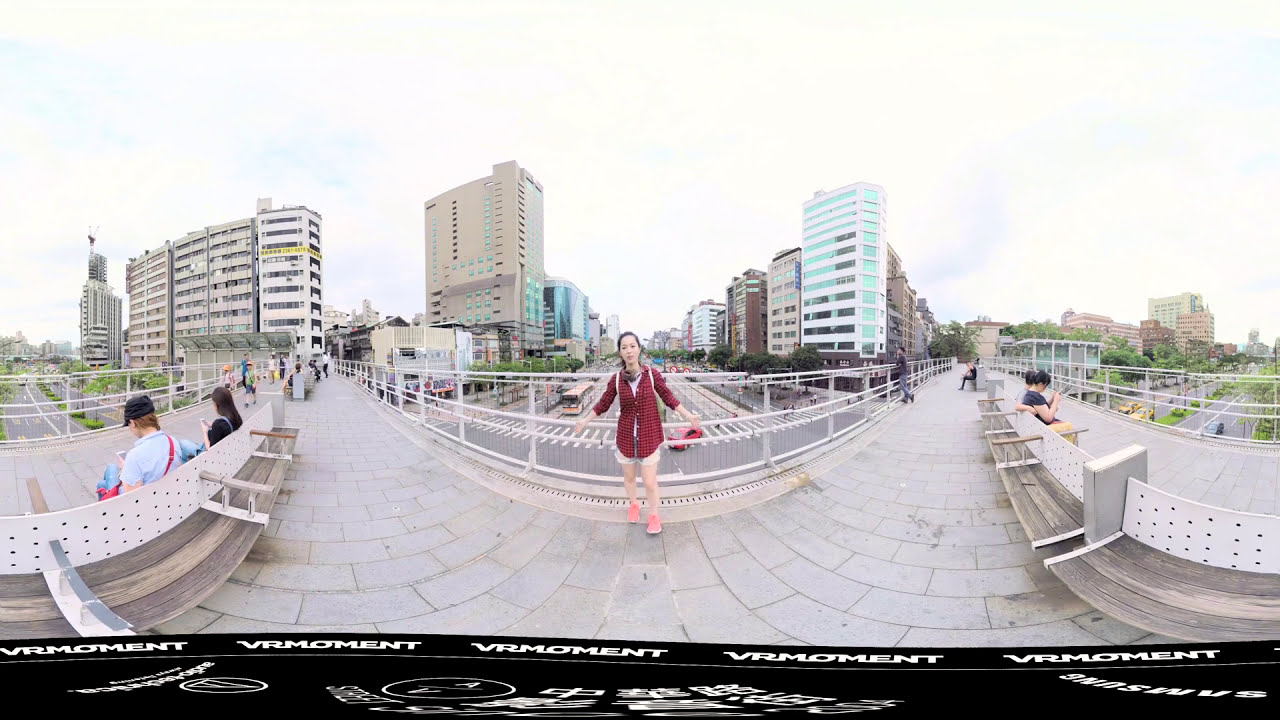The image captures a 360-degree panoramic view of a bustling cityscape centered around a pedestrian walkway that spans over a multi-lane road. A female figure, dressed in white shorts, a maroon or red flannel long-sleeve shirt, and pink shoes, stands posed with her arms outstretched, facing the camera, possibly wearing a backpack. She leans against a metal railing that runs along the tiled walkway. Flanking her on either side are white benches with brown wood seats, occupied by people either sitting or standing, enjoying the urban vista. The wide roadway below is marked with white lines, hosting multiple lanes of traffic including buses and cars. Tall, modern office buildings with glass panes and varied shades of beige, brown, and blue rise on both sides of the street, forming a canyon-like corridor. In the peripheral edges of the image, the road stretches further, bordered by patches of greenery and trees. The sky above is mostly white with a hint of blue. A black banner at the bottom of the image reads "VRMOMENT" in white text, alongside some symbols and an upside-down “Samsung” logo in the bottom right corner, emphasizing the virtual reality element of the photograph.